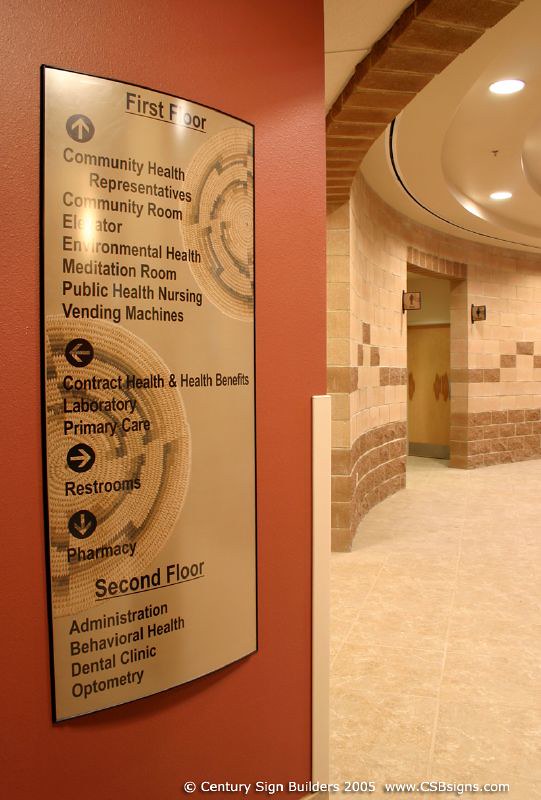The image depicts a detailed interior view of a public health building, showcasing the ground floor or basement area. Central to the image is a large directory sign, printed in black font, providing directions to various facilities within the building. The sign starts with an upward-pointing arrow labeled "First Floor," listing: community health representatives, community room, elevator, environmental health, mediation room, public health nursing, and vending machines. An arrow pointing left directs to contract health and health benefits, laboratory, and primary care, while a right-pointing arrow indicates the restrooms. Just below, a downward arrow directs to the pharmacy. In smaller font, "Second Floor" is listed, indicating administration, behavioral health, dental clinic, and optometry. The sign features a watermark at the bottom right: © Century Sign Builders 2005 (www.cbssigns.com).

Adjacent to the sign is an entrance to a restroom, indicated by male and female symbols on either side of the doorway. The floor is covered in stone-colored tiles, and the walls are constructed from a mix of tan and brown cinder blocks, forming a curved structure. The ceiling is adorned with a couple of metal light fixtures. This detailed layout provides clear navigation for visitors seeking various health services in the facility.